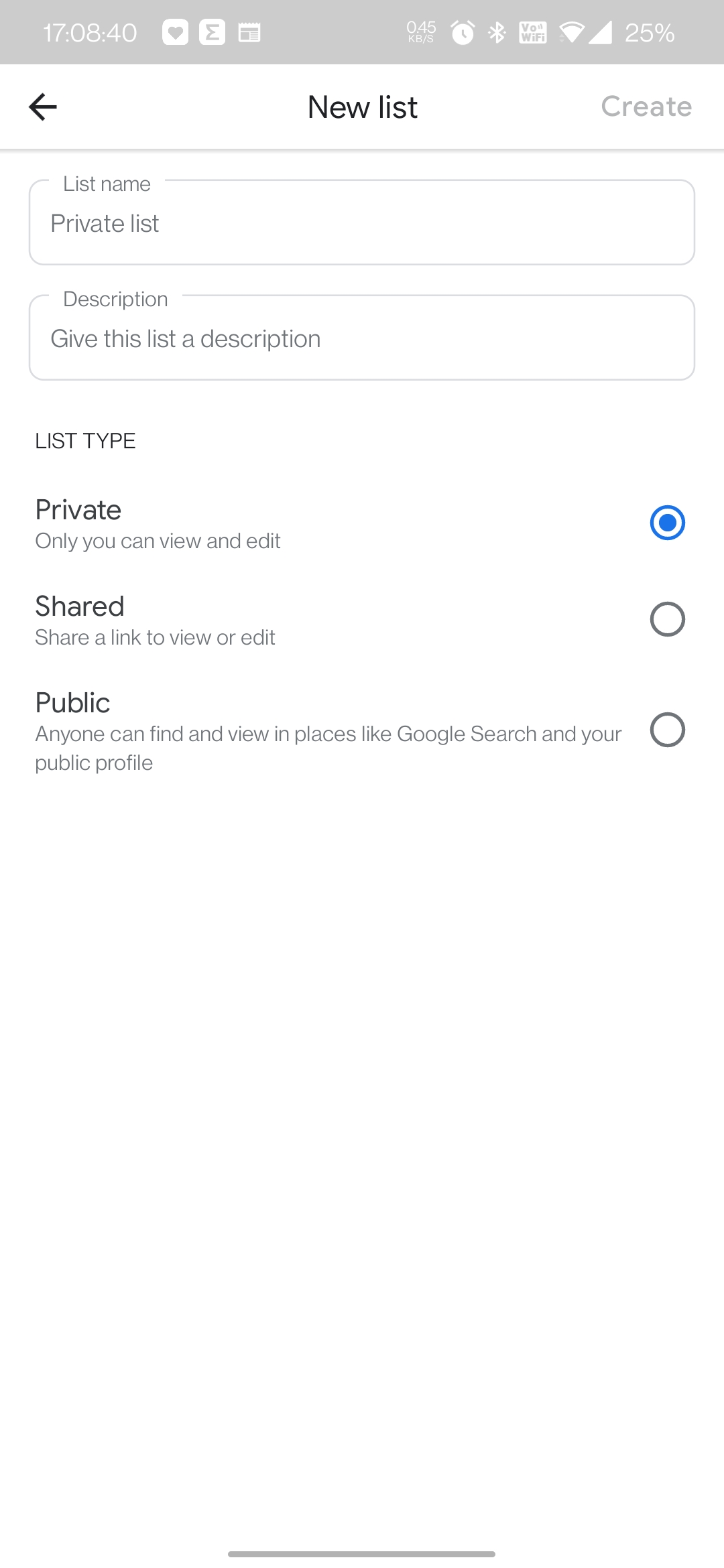Screenshot of a mobile device displaying an app interface for creating a new list. The time displayed is 17:08:40. In the status bar at the top, there are several app icons, signal strength, Wi-Fi status, a battery indicator showing 25% remaining, and other miscellaneous icons. The app header has a grey bar with the title "New List" in black, and the button "Create" in lighter grey on the right. Below, user input fields appear in lighter grey: "List Name," "Private List," "Description," and "Give this list a description.” Further down in black are the list type options: "Private" (selected), "Shared," and "Public." Each option has a brief description: "Private: Only you can view and edit," "Shared: Share a link to view or edit," and "Public: Anyone can find and view in places like Google Search, and your public profile." The background is predominantly white, contrasting with the grey bar at the top.